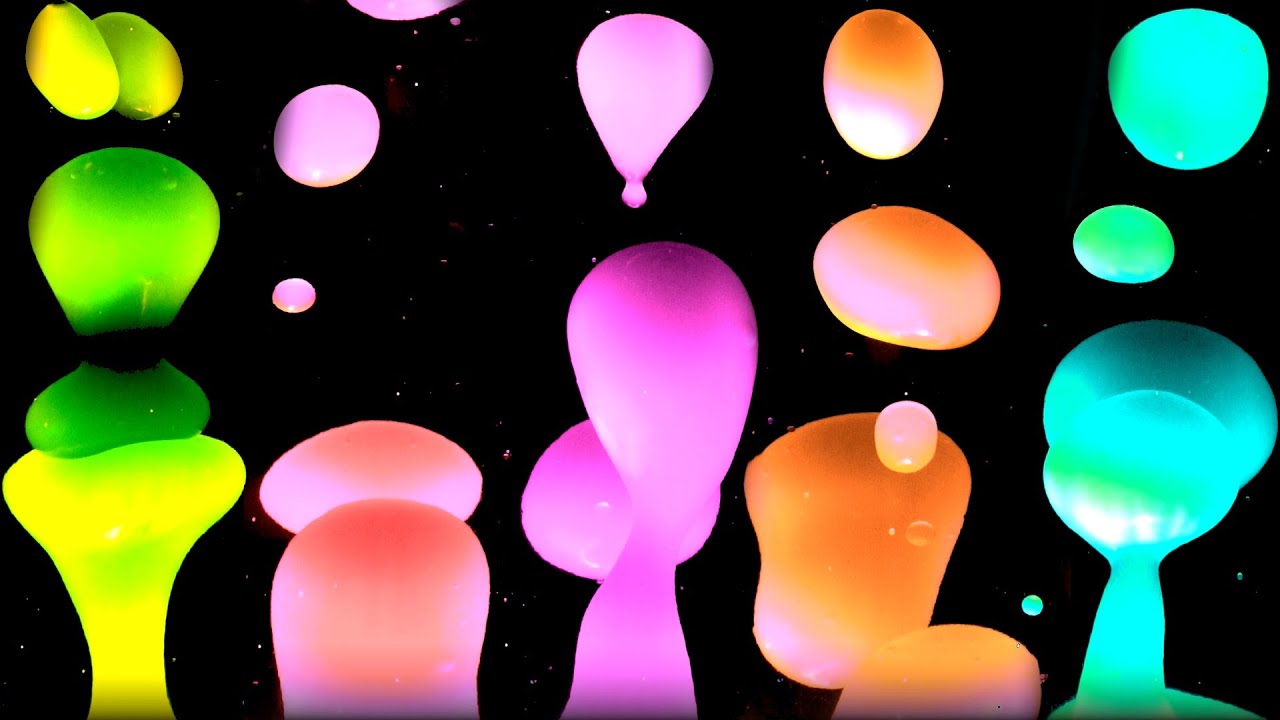The image depicts a rectangular photograph with a black background, reminiscent of viewing multiple lava lamps in slow motion. Starting from the left, there is a thick, bubbling liquid flowing upwards in shades of yellow, lime green, and pink. This transitions to a vibrant orangish-pink column in the middle, which consists of lumpy, pill-shaped orbs. The center features a prominent cluster of pink bubbles, followed by another orange column. Finally, on the far right, there are pillars of bluish-green and green, all creating a mesmerizing array of colorful, floating liquids resembling the graceful, undulating movement of lava lamps.